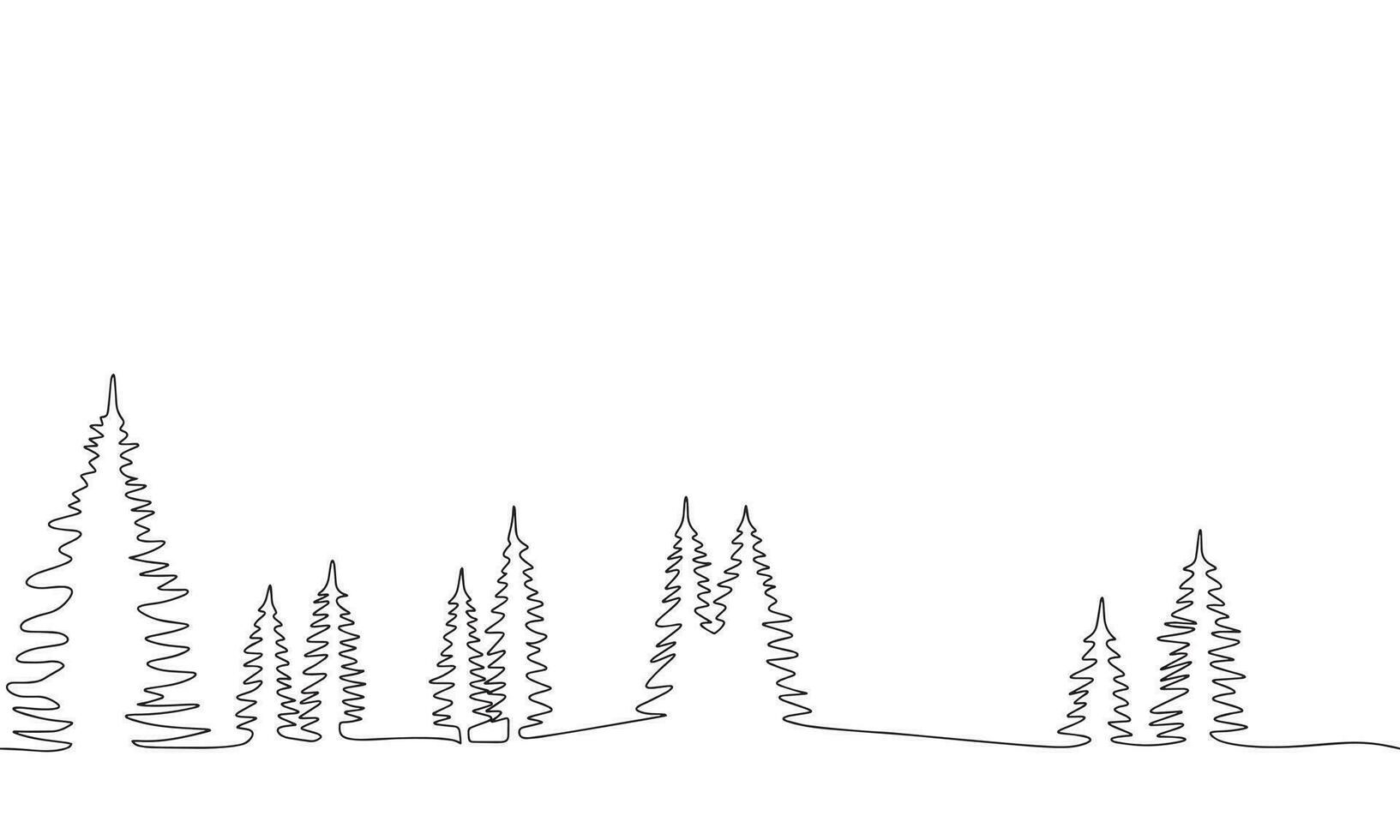The image showcases a series of stylized pine trees, all against a stark white background. These trees are created using a single, continuous black line that zigzags up and down to form the outline of the trees' branches. Starting from the bottom left, the line snakes its way across the canvas, depicting a sequence of nine pine trees.

The formation begins with a large tree on the far left, followed by two smaller trees grouped together. There's a noticeable space before another pair of smaller trees emerge, standing close to each other and similar in size to the first small pair. As the line progresses towards the right, it forms two more smaller trees, again closely spaced. Finally, the sequence ends with a solitary, larger tree on the far right.

The line traces a simple yet clever design, zigzagging vertically to create the illusion of branches and the characteristic pointed tops of pine trees. The entire ensemble has a minimalist, computer-drawn aesthetic, capturing the trees with fine precision and uniformity. This clever use of a single line to represent multiple trees highlights both artistry and technical skill, hinting at the potential for further development and possibly color in future iterations of the work.